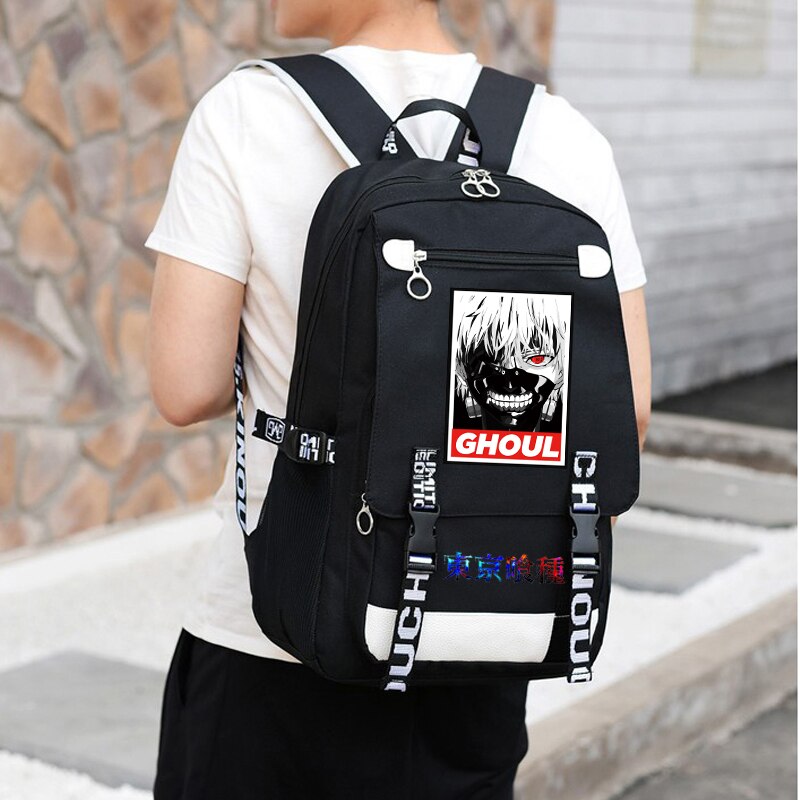In an outdoor setting, against a backdrop featuring a stone wall and a white garage door, a person—wearing a white T-shirt and black pants—models a pristine, black backpack. The main focus of the image is the backpack, which boasts a standout design. Central to the backpack is a striking illustration of a character from the Tokyo Ghoul anime, depicted with a black mask, exposed teeth, and a red eye. Below this illustration, the word "GHOUL" is prominently displayed in white within a red rectangle. The backpack features silver zippers and multiple black click straps, with one strap displaying the word "limited" in white. The bottom compartment of the backpack is adorned with intricate kanji characters. The straps, both over the shoulders and on the sides, are marked with large white text, enhancing the aesthetic appeal of this stylish, well-crafted accessory.